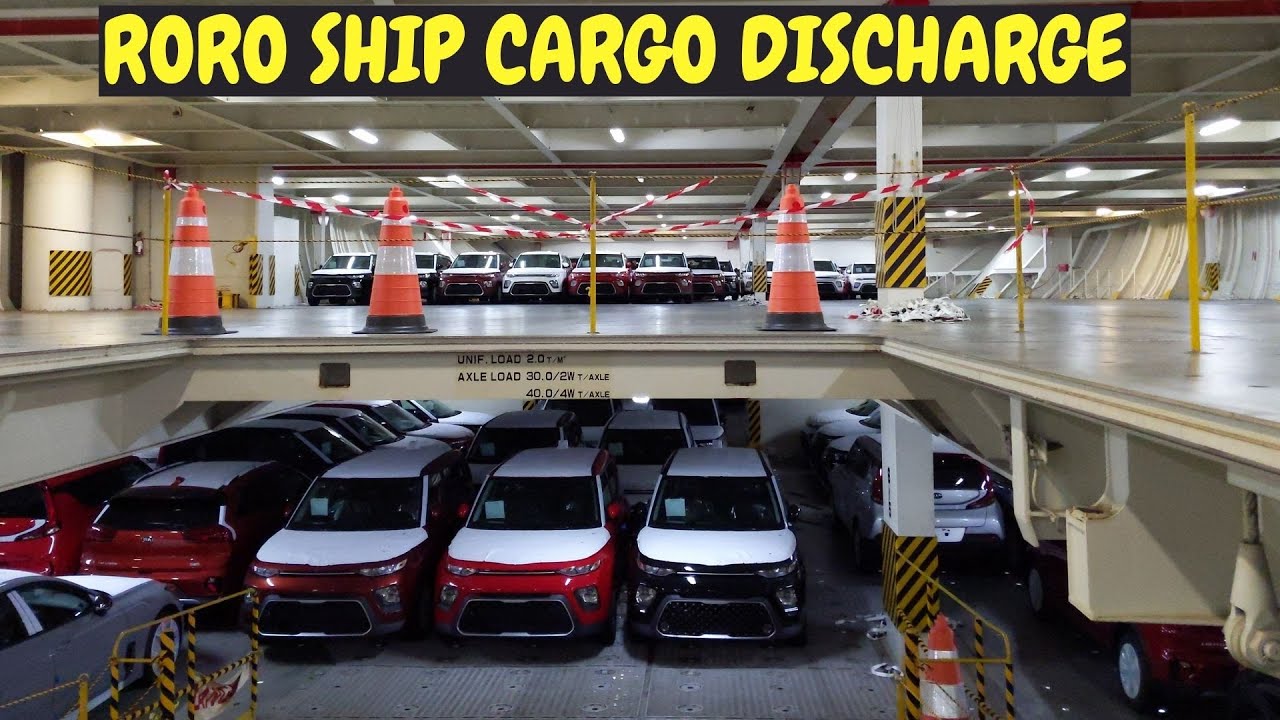This photograph captures the intricate interior of a RoRo ship, highlighted by a black banner with yellow text reading "RoRo Ship Cargo Discharge" at the very top center. The image reveals a two-layered cargo area designed to transport vehicles. The top layer features a shiny reflective gray surface with rows of neatly parked white and red cars towards the back. This upper deck also displays several orange and silver safety cones, yellow poles, and a thin brown rope demarcating the edges of a large rectangular hole that provides a view into the lower cargo area. The walls are painted red, and the ceiling is lined with various white support beams, along with tube lights illuminating the space. Additionally, on the side of a support column located to the right, there's detailed load information: “unified load, 2 tons per meter square,” along with specifications for axle loads indicating 2 WD and 4 WD capabilities, emphasizing its suitability for transporting a diverse range of vehicles.